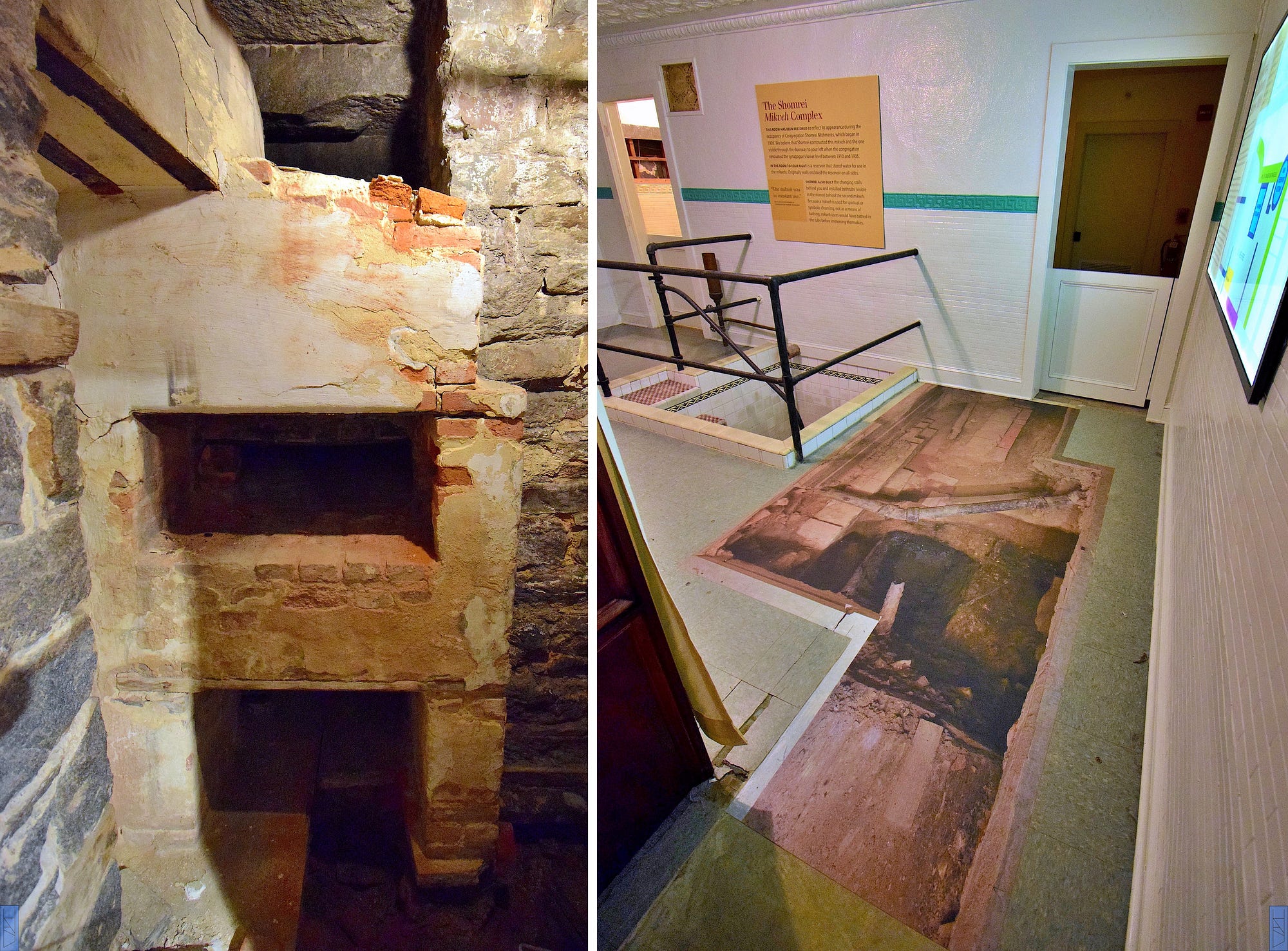The image is a broad horizontal rectangular frame, divided into two adjacent vertical rectangles. The left rectangle depicts a close-up view of a stone wall, possibly indicating an indoor, cellar-like setting with a rustic ambiance. The wall comprises stones of various shades, predominantly light and dark brown with some blue stones on the left side. The structure suggests the presence of a wood-fired oven or fireplace, characterized by rectangular openings reminiscent of a cooking area. This stone wall setting conjures an atmosphere that could be suited for a wine cellar or an underground bunker.

In contrast, the right rectangle portrays an interior scene that evokes a museum or gallery environment. This room features a juxtaposition of materials; the walls include sections of both brick and plaster. The stone floor is primarily light gray with interconnected rectangular patches of light and dark brown. Notable elements include a square opening in the floor against the far wall, safeguarded by black metal rails. Additional features include a yellow square sign with text on the wall and a door in the background, split into black and white segments. A staircase descends to a lower level, contributing to the multifunctional aspect of this space.